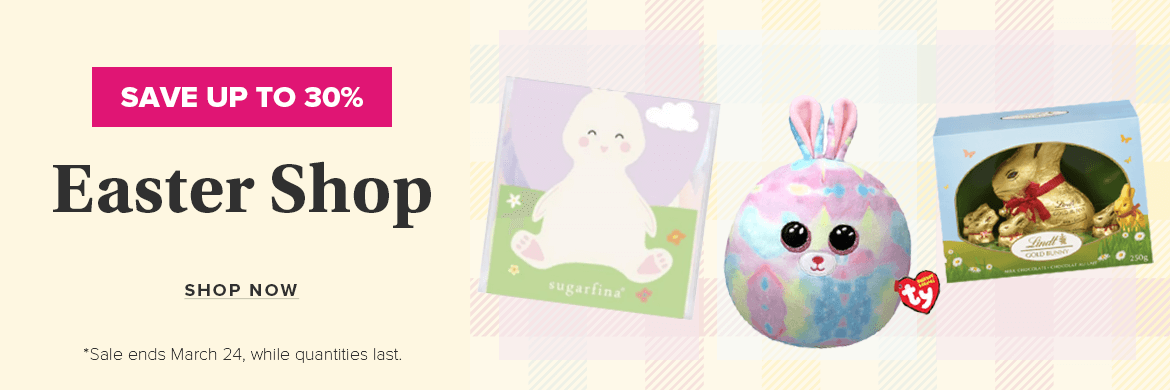The image features a promotional banner for Paige's Easter sale set against a light pale yellow, almost beige, background. In the upper left corner, a pink rectangular box contains white text announcing "Save up to 30%." Beneath this, bold black letters proclaim "Easter Shop," followed by a call-to-action in regular text stating "Shop Now." Below this, a notice reads, "Sale ends March 24th while quantities last."

To the right of the text, a playful plaid pattern of red, blue, and yellow stripes fills the background, adding a festive touch. Displayed in this section are three featured items: 

1. A book with a cover featuring a white rabbit sitting on a grassy green area.
2. A plush rabbit with a tie-dye pattern of pink, yellow, and blue, large round black eyes, and a red heart tag that reads "TY."
3. A large chocolate bunny encased in a blue box with a green grassy bottom, identified as "Lindell's Chocolate."

Each element combines to create an inviting and festive ambiance, perfect for attracting customers to Paige's Easter sale.